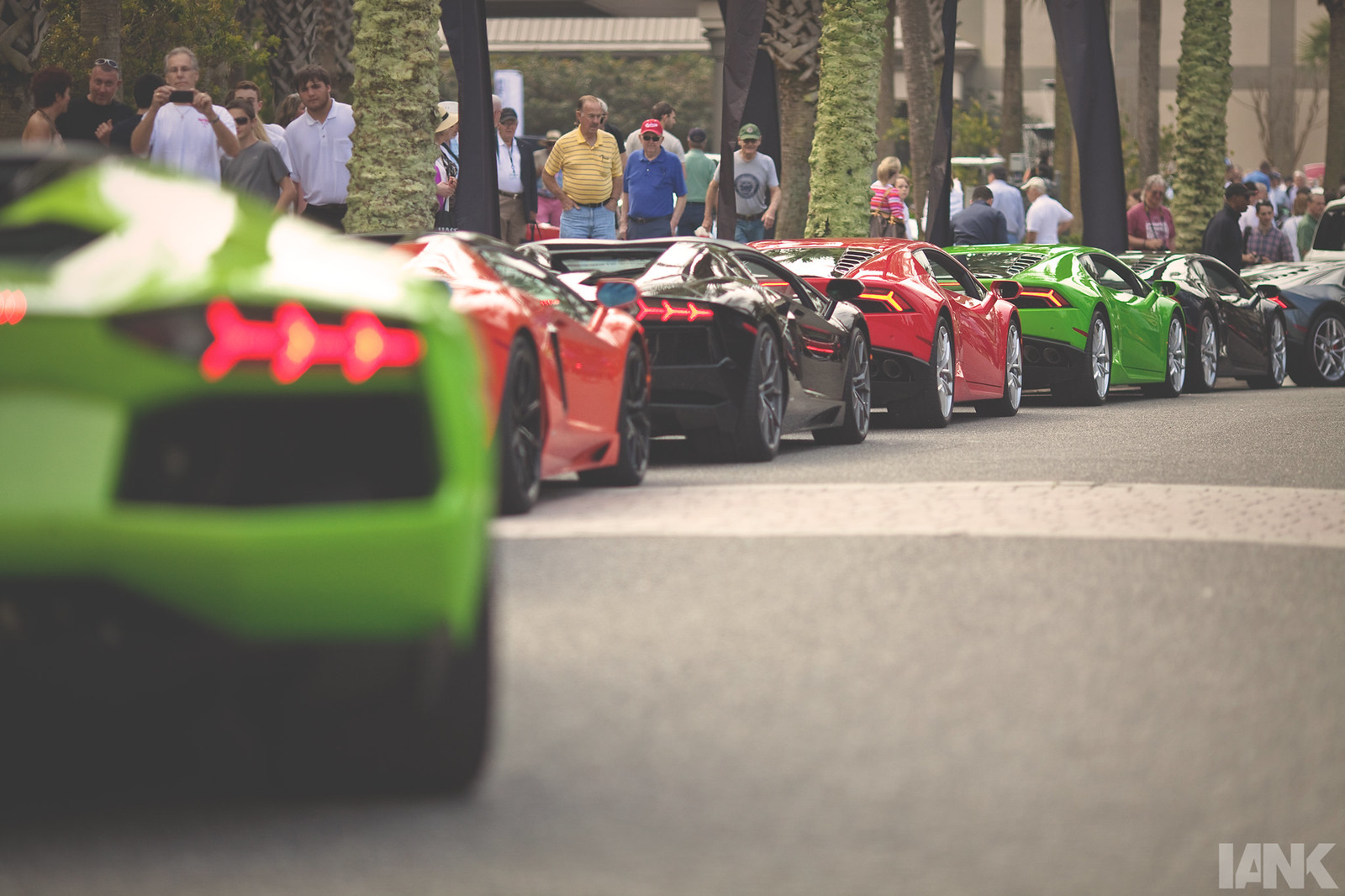The photograph, taken during the daytime, captures a low-angle view of a procession of sports cars driving in a curved formation from the left side of the image to the back, where they snake to the right. The cars, which include bright green, red, and black colors, are arranged one behind the other and display their striking features such as red brake lights and black tires with silver rims. The sports car closest to the camera is a vivid chartreuse green, though it is slightly out of focus, emphasizing the depth of the scene.

Along the left side of the image, towering palm trees with greenish bark provide a natural backdrop. Adjacent to these trees, on what appears to be a sidewalk, numerous onlookers can be seen. They are dressed in various colors, including white, denim blue, green, red, yellow, and maroon, and many are capturing the spectacle on their smartphones, admiring the vehicles. Near the top and left side of the image, a group of individuals is distinctly visible, detailed in their attire: a girl in a tank top, and various men in black, white, and gray shirts, with one man capturing the scene on his phone. At the bottom right, faint white letters "I-A-N-K" are transparent against the background, adding a subtle textual element.

Additionally, a tan and dark brown building stands behind the scene, partially visible amidst the crowd and the trees. This detailed composition, filled with vivid colors and dynamic human activity, highlights the enchanting allure of the sports cars in their vibrant outdoor setting.